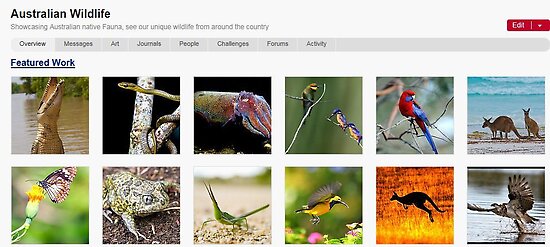**Screenshot of Desktop Displaying a Gallery of Australian Wildlife**

The image appears to be a screenshot taken from a desktop computer. The title of the gallery, "Australian Wildlife: Showcasing Australian Native Fauna," is prominently displayed in black font on a white background. This title encourages viewers to explore Australia's unique wildlife from across the country.

On the upper right-hand side, there is an "Edit" button with a red background and white letters, accompanied by a downward-facing caret indicating a dropdown menu. Below this button is a navigation bar with several categories listed in black font: "Overview," "Messages," "Art," "Journals," "People," "Challenges," "Forums," and "Activity." The "Overview" tab is currently selected.

Underneath the navigation bar, the subheading "Featured Work" is displayed in dark blue letters and is underlined, indicating it as the current section being viewed. Below this subheading, the gallery begins with two rows of thumbnails, each showcasing a variety of Australian wildlife.

### First Row of Thumbnails:
1. **Crocodile:** An image capturing the fierce demeanor of a crocodile.
2. **Snake:** A close-up of a snake, highlighting its scales and vibrant colors.
3. **Squid:** An underwater shot of a squid, showcasing its tentacles and fluid movement.
4. **Bird:** An unidentified bird species, perched elegantly.
5. **Parrot:** A vividly colored parrot, predominantly red and blue, sitting calmly.
6. **Kangaroos:** A pair of kangaroos, possibly a mother and joey, in a natural setting.

### Second Row of Thumbnails:
1. **Butterfly on a Flower:** A delicate butterfly resting on a brightly colored flower.
2. **Toad:** A toad perched on the ground, camouflaged amongst leaves and soil.
3. **Insect:** A close-up of an unidentified insect, highlighting its detailed anatomy.
4. **Bird in Flight:** A dynamic shot of a bird captured mid-flight.
5. **Kangaroo Jumping:** A kangaroo in mid-leap, illustrating its agility.
6. **Bird in Water:** A bird wading through shallow water, possibly looking for food.

This organized and visually appealing layout offers a comprehensive glimpse into the diverse and exotic wildlife found in Australia.